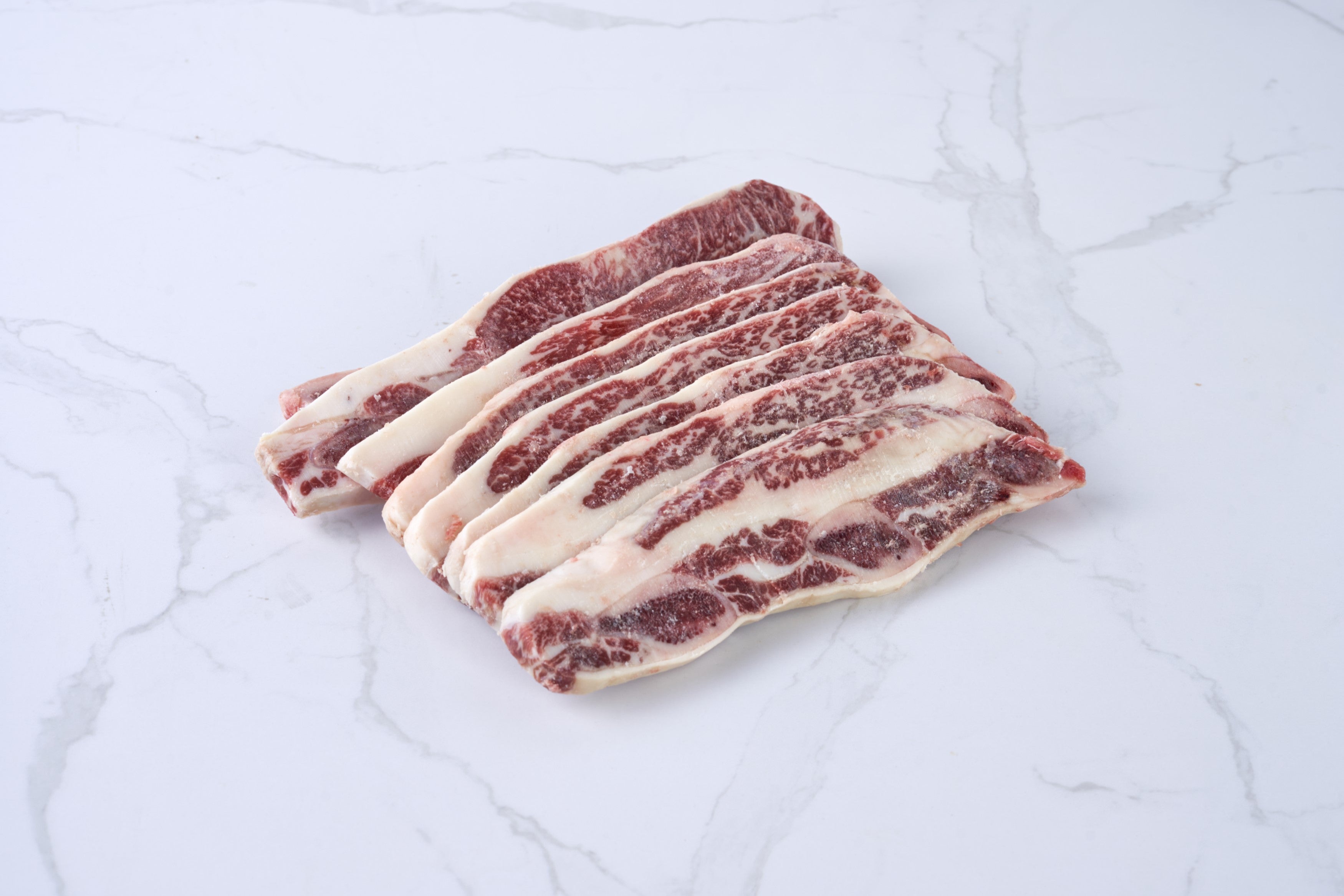The image displays a close-up view of seven to eight strips of meat, likely frozen beef short ribs, due to their rigid appearance and presence of ice particles. The meat, characterized by a rich reddish-brown color with substantial marbling, lies on a light white-gray marble countertop streaked with darker gray lines. Each strip features prominent veins of fat running through the meat, contributing to its high-fat content, typical of short ribs. The intricate marbling and clusters of white fat weave through the meat, especially noticeable towards the tops of the strips. The uniformity in the cuts suggests they originate from the same animal, though the exact type remains unspecified.